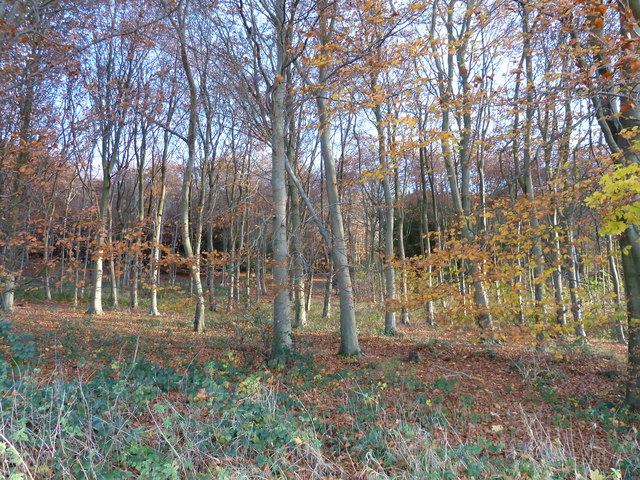This is a daytime image of a mature deciduous forest in late autumn. Dominated by tall, narrow-trunked trees ranging between 30 to 50 feet in height. The trees have mostly shed their leaves, which lie on the ground in various shades of brown and yellow, interspersed with patches of green grass and taller brown and green weeds. The barks of the trees are a light gray, almost white. In the background, the forest extends into another grove of darker green trees, while the upper part of the image reveals a blue sky with some white clouds visible through the sparse branches. The overall scene is tranquil and devoid of people or animals.